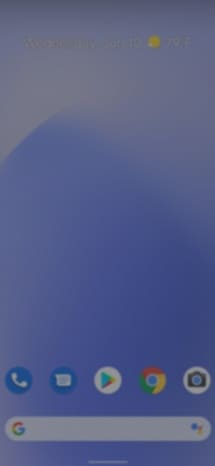A blurry, pixelated image displays a smartphone interface with a temperature reading of 9 degrees Fahrenheit in the sunlight. The top left corner features a white area, while various shades of blue are visible across the screen. The screen includes several recognizable icons, such as a phone icon, a message icon, the Play Store icon, the Google Chrome icon, and a camera icon. Additionally, there is a Google search bar with the iconic 'G' logo, accompanied by a Google Assistant feature. At the bottom is a navigation bar with different icons, all rendered in a somewhat pixelated manner.